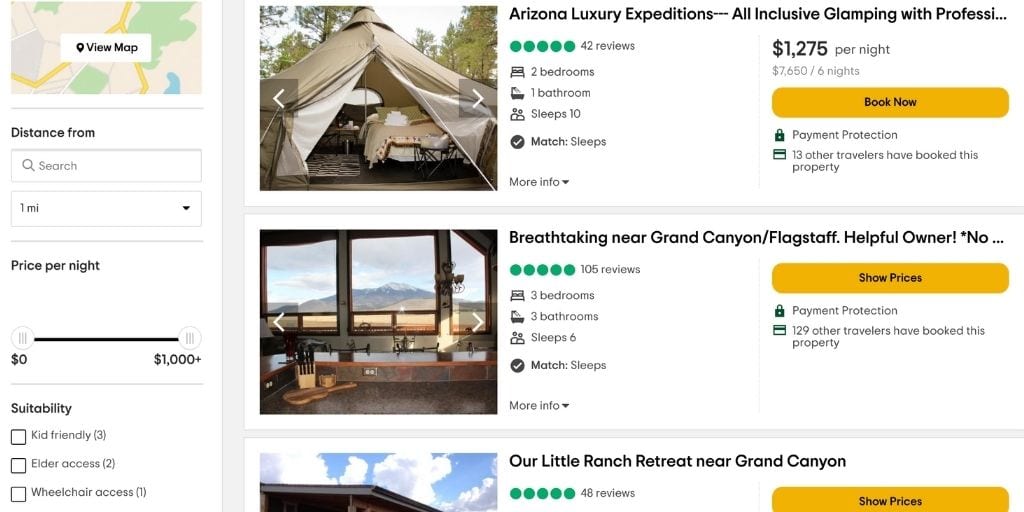This image is a screenshot from a travel website specializing in camping and hotel accommodations. In the top left corner, there is a small map with sections colored in green, yellow, and blue, with a "View Map" icon overlay. Below that, a search bar allows users to specify a distance range, with the option to filter by miles. The pricing filter ranges from $0 to $1,000 per night. Three suitability options are available for selection: kid-friendly, elder access, and wheelchair access.

The search results are partially visible, showcasing two and a half accommodation options. The first option features a large, tan yurt used for camping, with a visible bed inside, described as "Arizona Luxury Expeditions, all-inclusive glamping." The second option is an interior view of a hotel room looking out onto what appears to be the Grand Canyon, labeled "Breathtaking near Grand Canyon/Flagstaff, helpful owner." The third image is partially cut off, showing the top of a building shrouded in clouds, with the text "Our Little Ranch Retreat near Grand Canyon."